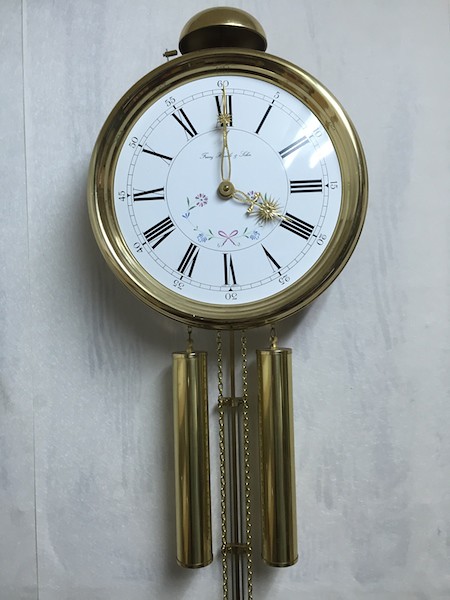The photo captures a wall-mounted clock set against a pale gray wallpaper backdrop. The wallpaper exhibits visible seams to the left of the clock, with a slight bubbling at one of the seams. The clock itself features a round silver casing and a white face adorned with delicate light blue floral designs and a small gray ribbon near the bottom. Atop the clock sits a bell, and elegant gold chimes dangle from the bottom. The slender hands, also gold in color, point to the time, which is approximately 4 o'clock. Faint black italic text is inscribed just beneath the number 12 on the clock face. A bright reflection from ceiling lights can be seen in the clock's glass cover.